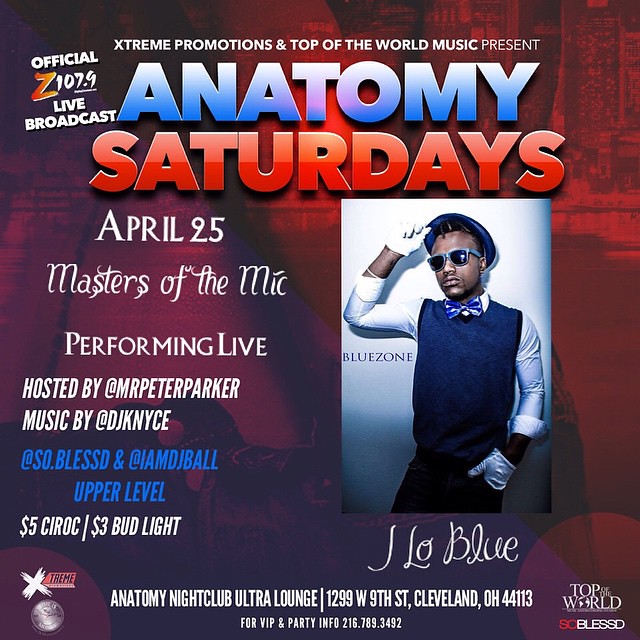The image is a colorful, square advertisement for an event at Anatomy Nightclub Ultra Lounge, located at 1299 West 9th Street, Cleveland, Ohio, 44113. The backdrop is a dynamic blend of red, blue, and purple, resembling a city skyline. The right side of the advertisement features a dark-complected gentleman standing against a white wall. He is dressed in a blue hat, blue vest over a long white shirt, blue bow tie, white gloves, black pants, and dark sunglasses, and he is tipping his hat while gazing towards the viewer. In elegant script beneath his image, it reads "JLo Blue," and next to him, the words "Blue Zone" are displayed.

At the top, the text announces, "Extreme Promotions and Top of the World Music Present," followed by "Anatomy Saturdays" in vibrant red. The official Z107.9 live broadcast is indicated in the upper left. The event is scheduled for April 25th and is titled "Masters of the Mic Performing Live." It will be hosted by Mr. Peter Parker with music by DJ Nice, So.Blessed, and I am DJ Ball, taking place on the upper level. Drink specials are listed as "$5 CIROC" and "$3 Bud Light." At the bottom, for VIP and party information, the contact number is 216-789-3492.